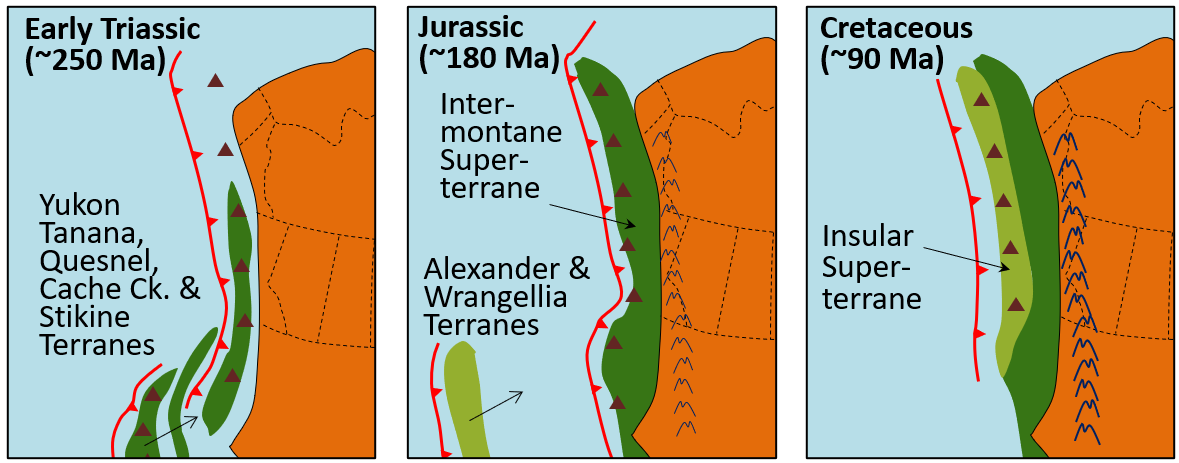Illustrated educational diagram showcasing geological changes from the Early Triassic to the Cretaceous periods. The image is comprised of three vertically rectangular panels, each bordered with a thin dark line and separated by horizontal white space. Each panel has a light blue background with black text detailing different eras and associated geographies.

From left to right:

1. **Early Triassic (250 MA)**
   - With text mentioning "Yukon, Tanana, Quesnel, Cache Creek, and Stycane Terrains."
2. **Jurassic (180 MA)**
   - Highlighting "Intermontane Superterrane, Alexander, and Wrangellia Terrains."
3. **Cretaceous (90 MA)**
   - Indicating "Insular Superterrane."

The panels collectively illustrate the transformation of the land over a span of millions of years, emphasizing geological and biological changes during these key periods in Earth's history.